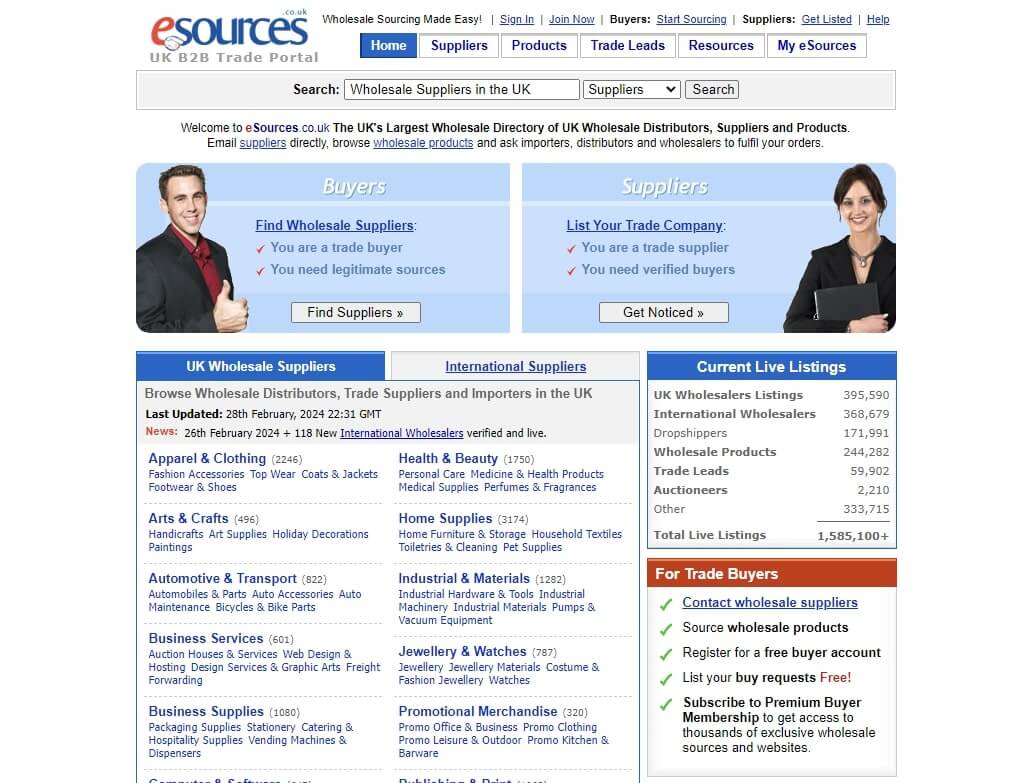A detailed screenshot of a wholesale supplier's website features a predominantly white background with blue and black text. The top left corner displays the site's logo, "eSources," with the tagline "UK B2B Trade Portal." To the right, a home button has been clicked, showcasing the homepage. Beneath this, a search bar is visible where a user has entered the query, "wholesale suppliers in the UK."

Two blue boxes dominate the central portion of the screenshot. On the left, there is an image of a white man with dark hair, wearing a dark jacket and red shirt. This box is labeled "Buyers," and it includes the tagline "Find wholesale suppliers. You are a trade buyer. You need legitimate sources." Below, a call-to-action button reads "Find Suppliers."

The blue box on the right features an image of a young white woman with dark hair, wearing earrings, a dark shirt, and a necklace, hugging a binder. This box is labeled "Suppliers," alongside the text, "List your trade company. You are a trade supplier. You need verified buyers." It also includes a call-to-action button labeled "Get Noticed."

The lower part of the screenshot contains a list of UK wholesale suppliers. The user has clicked on "UK Wholesale Suppliers," though an option for "International Suppliers" is also available but not selected. This section features multiple categories including Apparel and Clothing, Arts and Crafts, Business Services, Home Supplies, and Jewelry and Watches, among others.